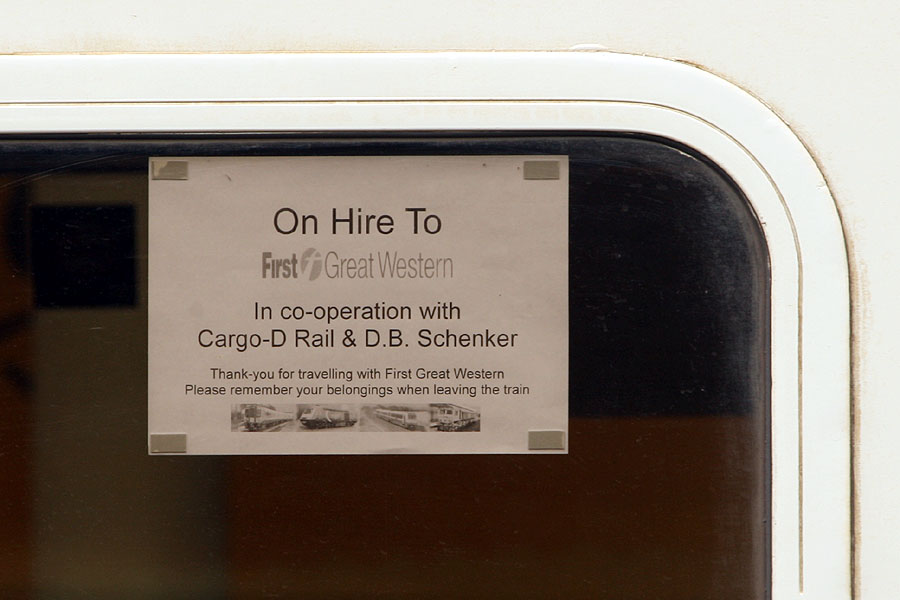This photograph shows a slightly dirtied, aged-framed window of a passenger train, offering an exterior view. Taped to the glass on the inside of this window is a horizontally-oriented, postcard-sized sign on white paper with centered black text. The sign, framed by the window, includes a message from the train operators, which reads: "On hire to First Great Western in cooperation with Cargo D Rail and DB Schenker. Thank you for traveling with First Great Western. Please remember your belongings when leaving the train." Below this text, there is a series of four small photographs depicting various trains. The sign serves as a reminder for passengers to collect their belongings before disembarking.